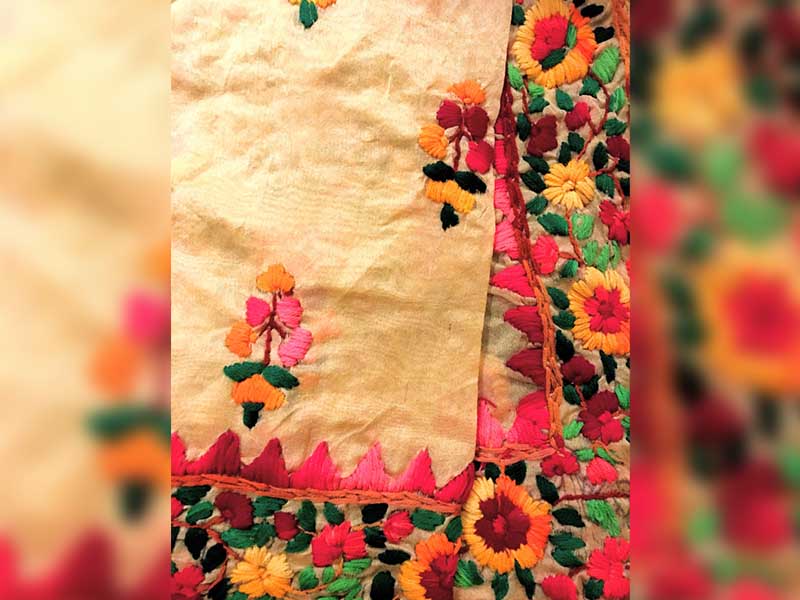The image is a close-up photo of a colorful piece of fabric, possibly a blanket, showcasing intricate floral embroidery. The fabric is split into two distinct sections: the left side is mostly yellowish-tan adorned with orange, pink, and green tile-patterned plants, while the right side is a darker gray featuring vibrant yellow, pink, and red flowers. Both sections are bordered with an intricate orange design embellished with pink triangles pointing inward. The embroidered designs on the fabric are rich in detail and color, incorporating bright hues like orange, yellow, pink, red, and green, with the floral patterns including elements that resemble daisies and other stylized blooms. The old-fashioned or vintage appearance of the fabric suggests it has a touch of timeless craft. In the background, blurred yet similarly colorful tones—orange and yellow—echo the vivid palette of the main fabric, enhancing the overall intricate and vibrant aesthetic.